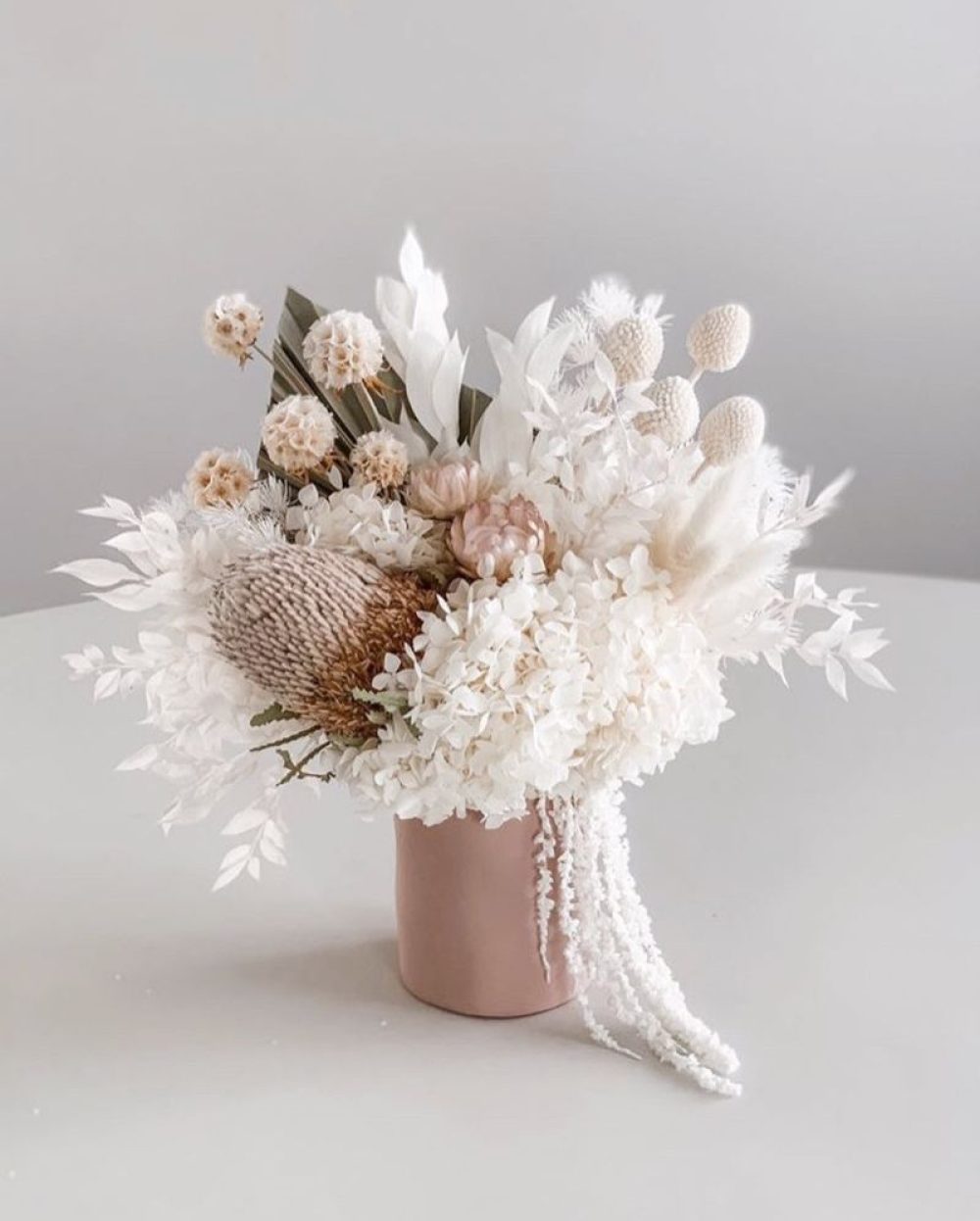This image features a beautifully arranged floral centerpiece situated on a white table. The centerpiece is housed in a light pinkish-peach vase, which complements the soft color palette of the flowers. The floral arrangement predominantly consists of white flowers of various kinds, including fluffy, carnation-like blooms. Interspersed among the white flowers are delicate light pink and peach blossoms, adding subtle hints of color. Some tendrils and white leaves cascade down from the arrangement, even touching the table. The background is a soft gray, enhancing the pastel hues of the flowers and the vase. This delicate and enchanting floral arrangement, with its bridal-like appearance, suggests it might be used as a wedding table centerpiece, embodying an elegant and romantic aesthetic.